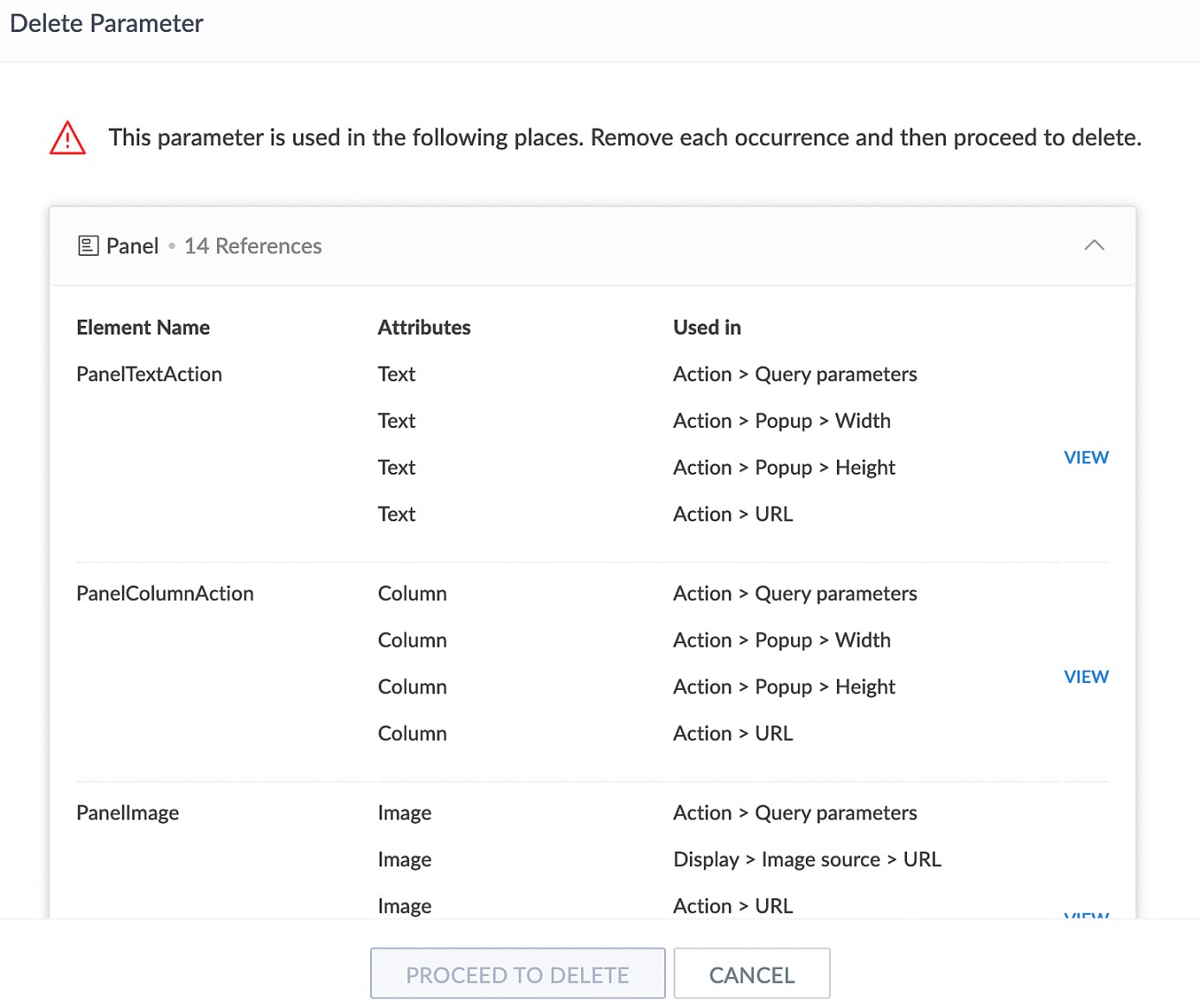The image appears to be a screenshot from an application or website interface displaying a warning and usage summary for deleting a specific parameter. 

At the top left, black text reads "Delete Parameter." Below this heading is a red-outlined triangle with a red exclamation mark in the center, signaling a warning. Next to the triangle, a message states, "This parameter is used in the following places. Remove each occurrence and then proceed to delete."

Under this message is a rectangular box titled "Panel" beside a small square logo and the text "14 references." Beneath the header section, the box is divided into three columns: "Element Name," "Attributes," and "Used In."

- The "Element Name" column lists the following items:
  1. Panel Text Action
  2. Panel Column Action
  3. Panel Image

- The "Attributes" column corresponds with each element name and includes values:
  1. Text
  2. Column
  3. Image

- The "Used In" column provides the context for each element's usage:
  1. Action (associated with 'Query Parameters' and the word "View" in blue text on the right)

At the bottom of the screenshot, there are two buttons: a grayed-out "Proceed to Delete" button and a white "Cancel" button.